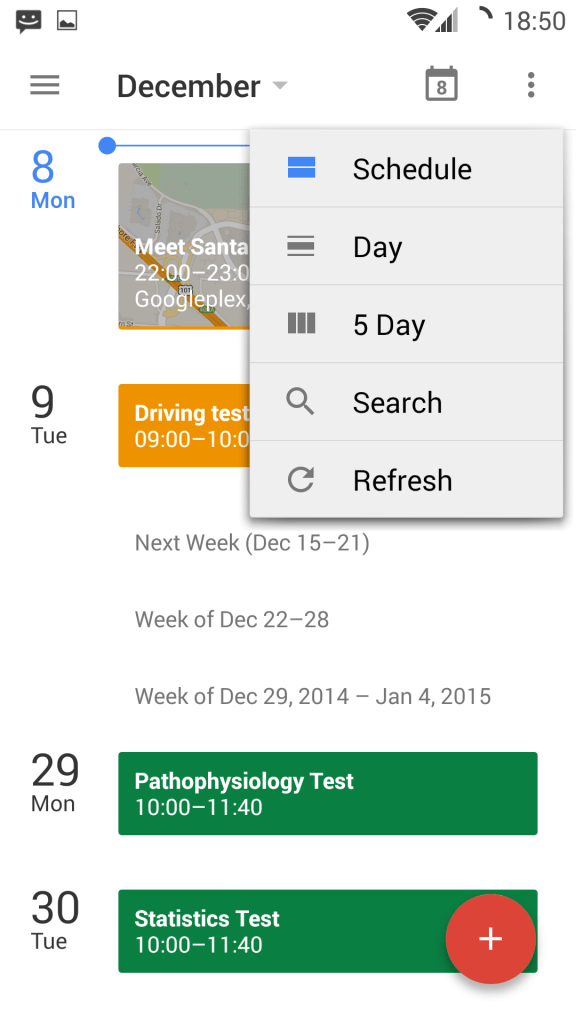In the image, an individual is viewing their December calendar on their phone. The interface displays "December" prominently at the top, with a small calendar emoji and a set of three dots to the right. In the top-right corner, the time reads 18:50, and the status indicators show a Wi-Fi connection and a battery level at 75%. On the left side of the screen, there's a smiling dialogue emoji followed by an image. Below this section, three grey bars are visible, with another "December" in black to their right, accompanied by a drop-down box, which appears to have been clicked.

The calendar view is set to a specific day, Monday the 8th, highlighted in blue. The details of the day's schedule are partially obscured by a dialogue box which includes options such as "Scheduled Day," "Five Day Search," and "Refresh." However, it is discernible that there is a meeting scheduled with Santa from 22:00 to 23:00, to take place at the Googleplex, which is also displayed on a map.

Further down, Tuesday the 9th is listed, marked in black, indicating it is not currently selected. One of the events for that day is a driving test scheduled from 9:00 to 10:00, enclosed in an orange box, followed by three other events.

The calendar also includes additional weekly views: December 15th to 21st, December 22nd to 28th, and December 29th to January 4th. For Monday the 29th, there is a pathophysiology test from 10:00 to 11:40, highlighted in a green box. Similarly, on Tuesday the 30th, there is a statistics test from 10:00 to 11:40, also highlighted in green. Overlaid on the right side of the statistics test event, there's a plus icon encircled in red.